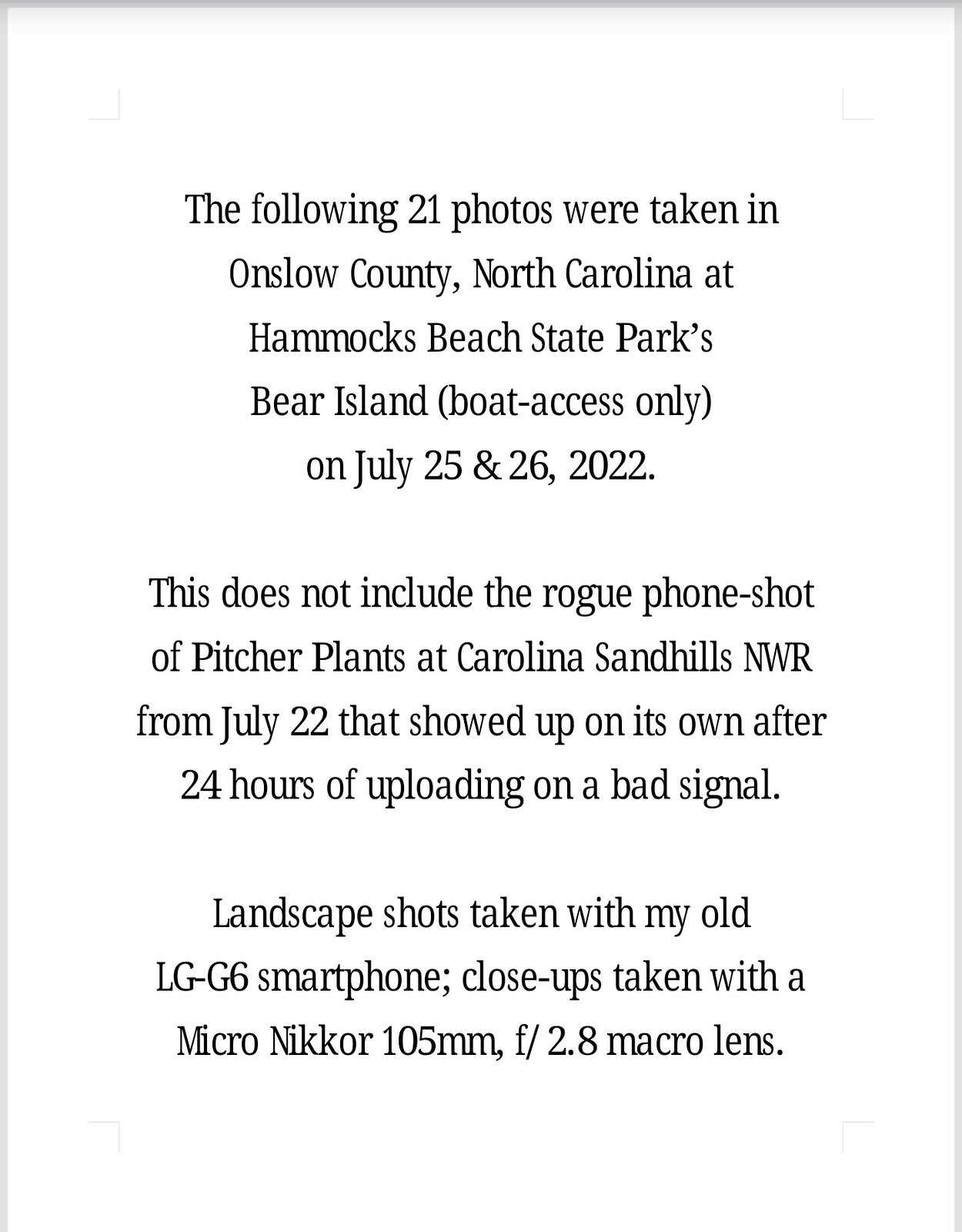The image features a white piece of paper with black text centered on it, bordered by a light gray edge. The text details the contents of a photographic collection, specifying that 21 photos were taken in Onslow County, North Carolina, at Hammocks Beach State Park's Bear Island, which is accessible only by boat. These photos were captured on July 25th and 26th, 2022. The note explicitly excludes a rogue phone shot of pitcher plants at Carolina Sandhills National Wildlife Refuge (NWR) from July 22, 2022, which appeared after a delayed upload due to a poor signal. The landscape shots were taken using an old LG G6 smartphone, while the close-up shots were captured with a Micro NIKKOR 105mm f/2.8 macro lens. The entire description is presented in black text against the white paper background.